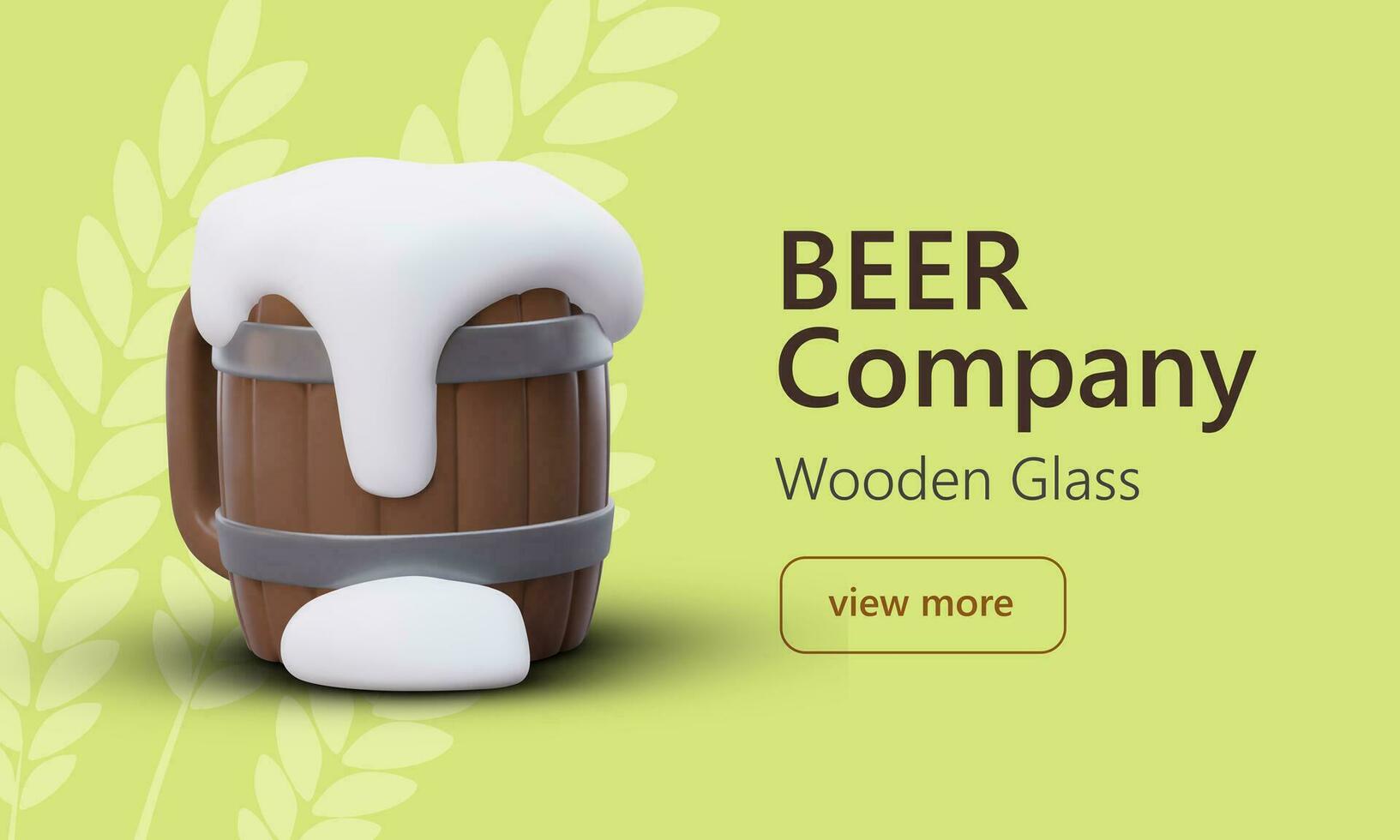The image is a horizontally-oriented advertisement for a generic beer company, featuring a 3D rendition of a barrel-type beer mug. This brown mug, designed to resemble a wooden stein, has two silver circular rings—one near the top and one near the bottom—and a handle. White foam from the beer overflows the top, with some foam dribbling down the side of the mug. The background is a light green with three lighter green strips depicting barley or oats. To the right of the mug, in dark brown text, is the phrase "Beer Company", followed by "Wooden Glass" in black text underneath. There is also a rectangular oval button in brown with the call-to-action text "View More". The image has a smooth, plastic-like appearance with soft edges.